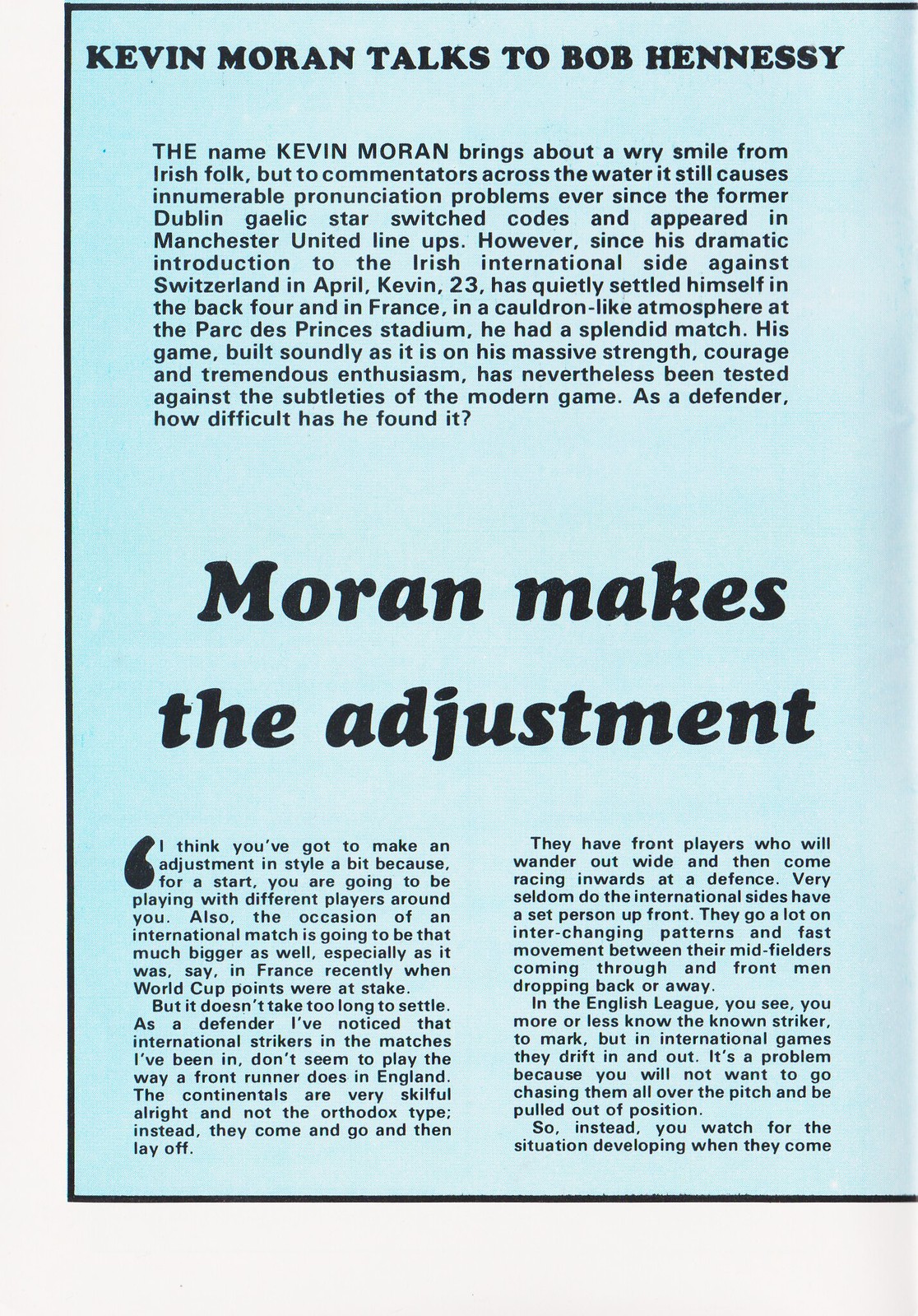This image features a page from a magazine with text discussing the Irish footballer Kevin Moran. At the top, it introduces the article with the headline, "Kevin Moran talks to Bob Hennessy." The article details how Kevin Moran's name evokes a wry smile from the Irish but presents pronunciation challenges for commentators abroad. It discusses Moran's transition from Dublin Gaelic football to playing for Manchester United, noting his appearances in the Manchester United lineup and his significant performances for the Irish international team, including a prominent match in France during World Cup qualifiers. The page has a blue background with black text, framed with a black outline on the top, left, and bottom edges. Midway through, there is a bold segment titled "Moran Makes the Adjustment," quoting Moran on the necessity of adapting his playing style due to different teammates and the grandeur of international matches. The detailed narrative highlights his strength, courage, and enthusiasm, and it concludes with reflections on his successful adaptation despite the challenges posed by modern football.